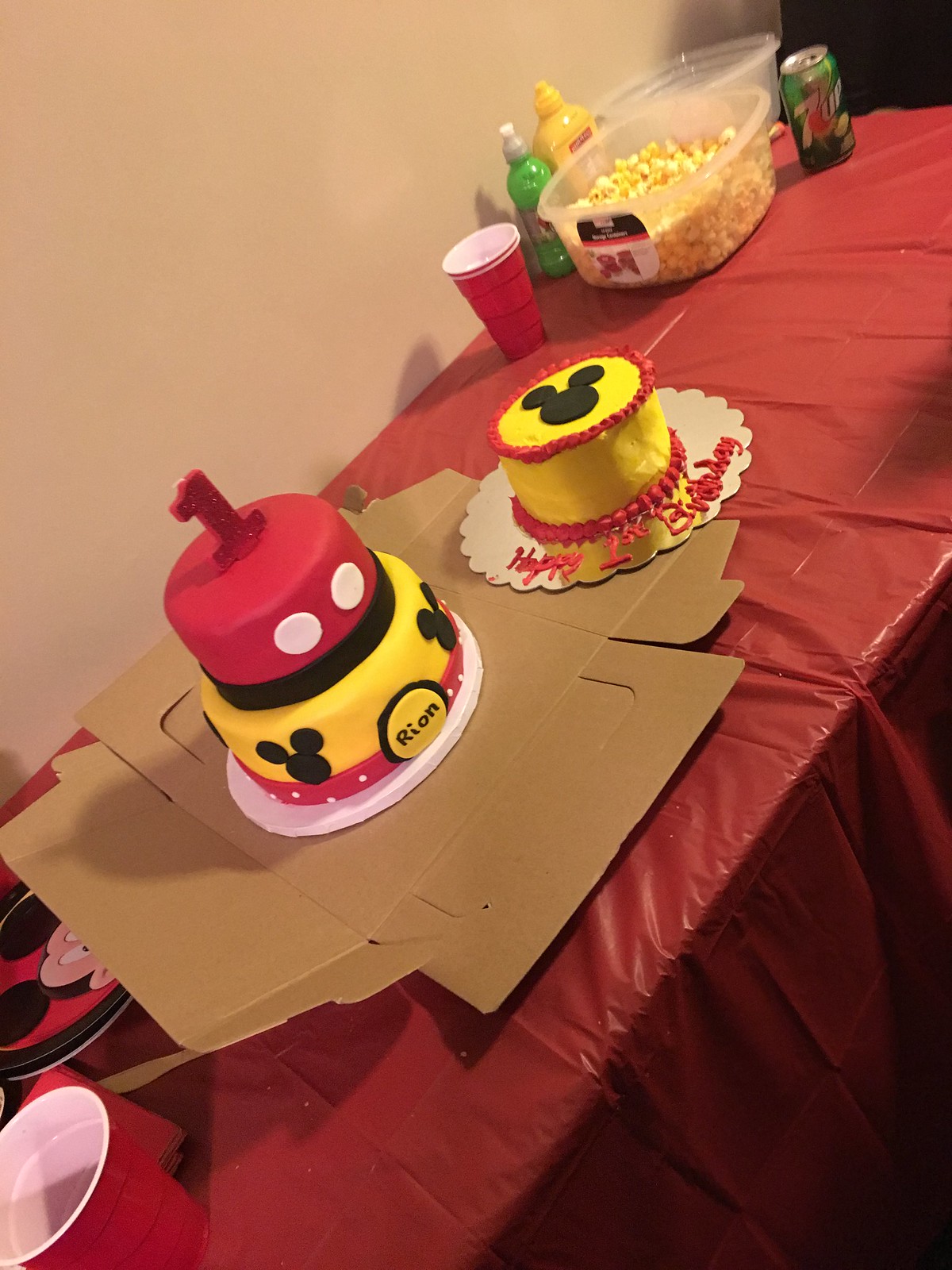The photograph captures a vibrant and festive birthday party setup for a little boy named Rian, who is turning one year old. The image is taken from an angled perspective, presenting the table, which is adorned with a red plastic tablecloth, running diagonally from the bottom left to the top right. Dominating the scene are two Mickey Mouse-themed cakes. The larger, two-tiered cake on the left features a yellow bottom layer adorned with black Mickey Mouse heads, a red border with white polka dots, and a round fondant emblem stating "Rion" in the center. The top tier is primarily red with white polka dots and a black border, capped with a sparkly number one candle. To the right is a smaller, single-tier yellow cake with red icing accents and a Mickey Mouse head on top, positioned on a tray that reads "Happy First Birthday" in red frosting. Surrounding the cakes are red Solo cups, Mickey Mouse-themed plates, a bowl of popcorn, and a 7-Up bottle, all contributing to the lively atmosphere of Rian’s first birthday celebration.